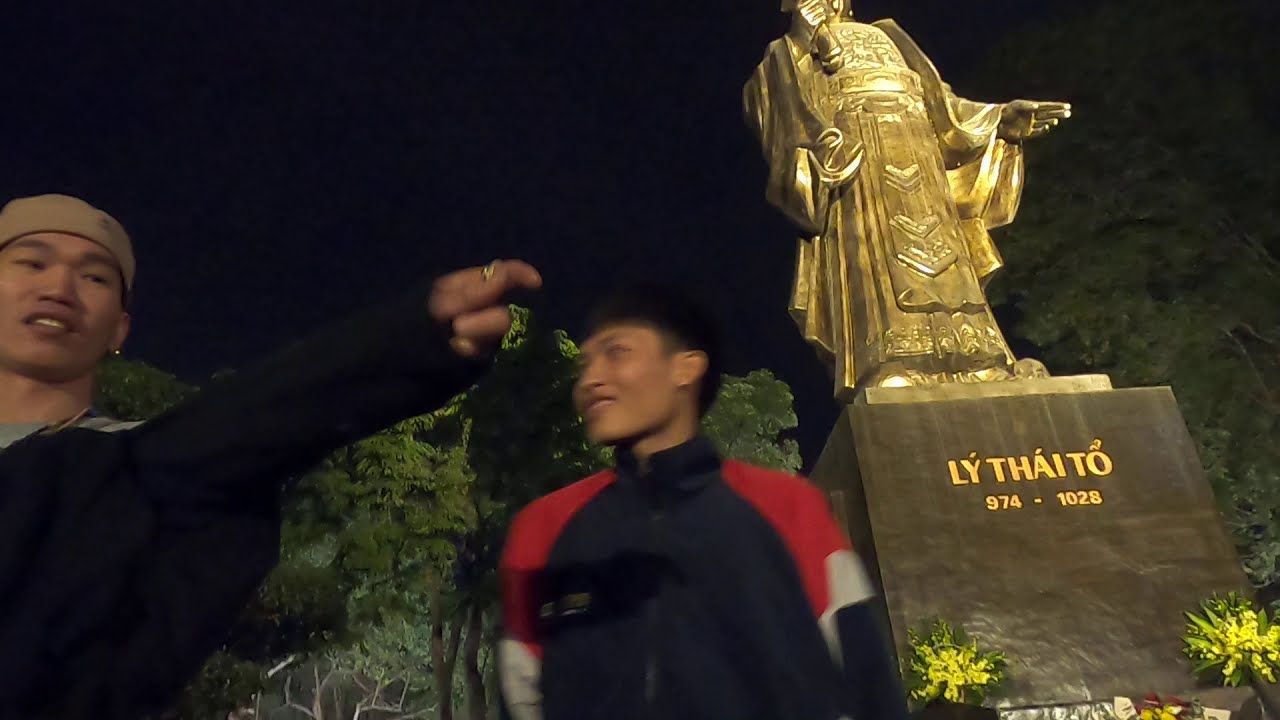In this outdoor nighttime scene, two young Asian men stand to the left and in front of an imposing gold-colored statue. The statue, which is missing its head from the top of the frame, is mounted on a large dark brown or gray granite base inscribed with the name "Lý Thái Tổ" and the dates "974-1028." This figure, dressed in intricate and ceremonial robes, holds a scepter or scroll in its right hand while extending its left in a blessing or pointing gesture. The base of the statue is surrounded by lit-up yellow-green plants, adding a mystical glow to the scene.

The two men pose confidently in front of the statue. One, to the center left, dons a black jacket with red and white detailing on the shoulders and is gesturing with his left arm extended, his finger pointing downward. The other, standing closer to the left edge, sports a black and red sweatshirt and a backward baseball cap, smiling with an earring visible in his left ear. In the backdrop, trees illuminated by ambient lighting frame the night sky, completing this striking, culturally rich image.